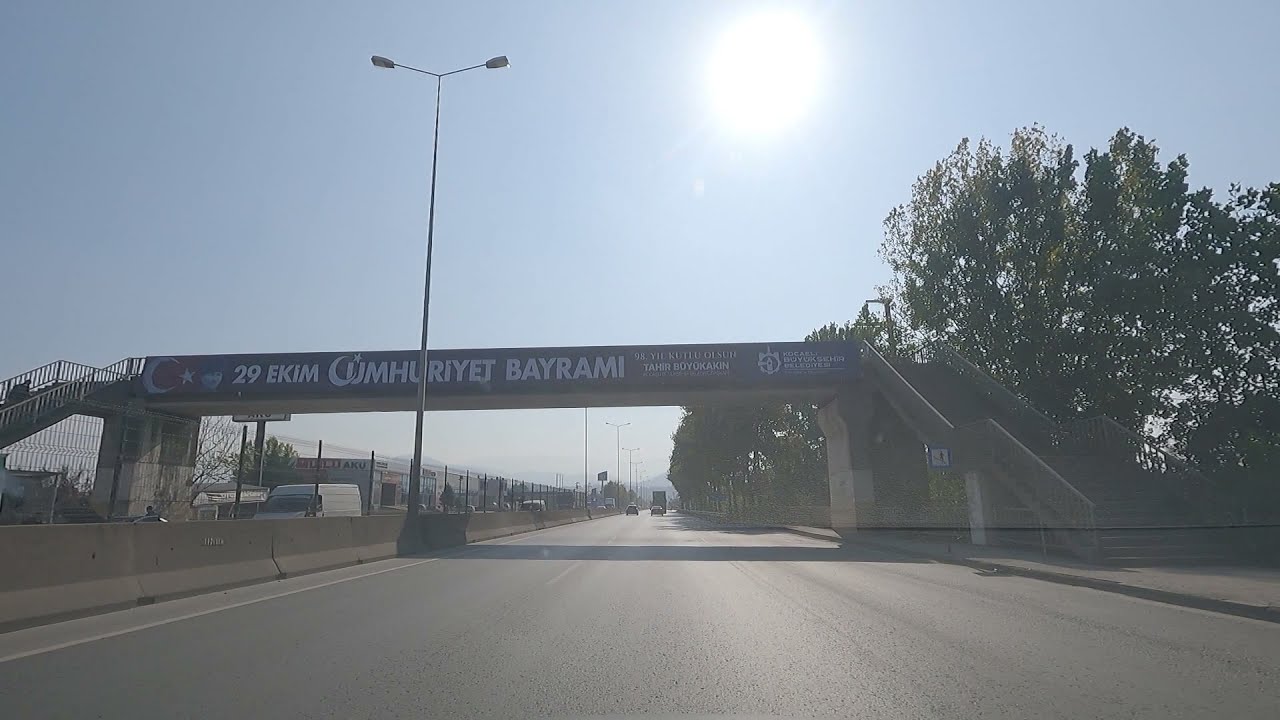This color photograph captures a sunny, bright summer day on a wide, mostly empty highway that stretches into the horizon. Dominating the scene is a pedestrian bridge arching over the road, adorned with a dark blue banner featuring white text in a foreign language, including "29 EKIM CUMHURİYET BAYRAMI." The bridge is accessible via staircases on both sides. To the right, dense, leafy green trees add natural beauty, while an overhead floodlight is positioned to the left of center. The road below is divided by concrete barriers and high metal fences, with a sparse number of cars and trucks visible, emphasizing the open and serene atmosphere of the roadway. The photograph appears to be taken from within a vehicle, providing a direct view of this scenic and structured landscape.